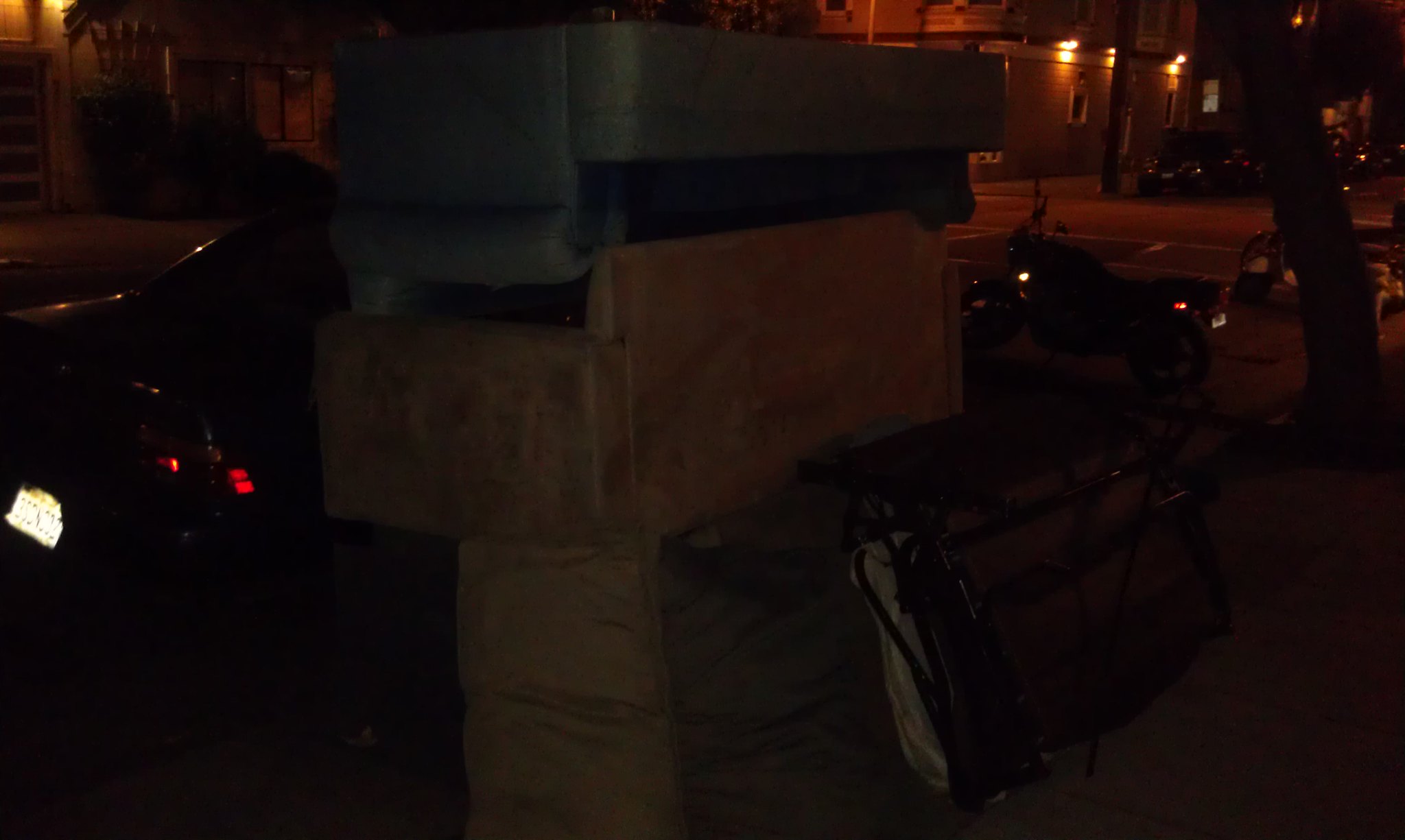The night scene in the photograph is taken from a vantage point that could be someone's porch, giving a view of a dimly lit suburban residential neighborhood. The image captures a small portion of a street with a car and a motorcycle parked curbside, both lightly illuminated, possibly by the flash of the camera or ambient street lights. The car's taillights and license plate are visible. Perpendicular to the car, a motorcycle is stationed. The foreground prominently features a stack of discarded furniture, including approximately four or five couches of various colors and positions—one gray couch inverted on top, a beige couch upright beneath it, and a couple more overturned ones interspersed with what might be a metal-framed item, possibly a fold-out bed. 

To the right of this stack of furniture, a tree is visible, planted close to the sidewalk. The background reveals buildings across the street, which appear to be at least two stories high and illuminated by orange side lights, resembling a storefront with upper-level apartments. Additional cars are parked further down the street past an intersection. The overall scene is dark, dreary, and gives a sense of an ordinary neighborhood at night, highlighted by the oddity of discarded furniture awaiting pickup or scavenging.